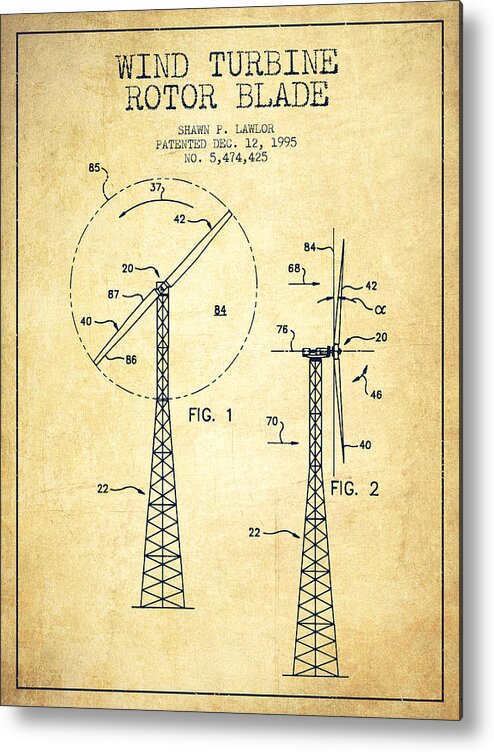This is a highly detailed patent diagram for a wind turbine rotor blade, submitted by Sean P. Lawler and patented on December 12, 1995, under patent number 5,474,425. The diagram is presented on a parchment-style background characterized by a weathered texture with varying shades of yellow and a thin black line border slightly inset from the edge. At the top, worn serifed black text reads "Wind Turbine Rotor Blade," followed by smaller text with the inventor’s name, patent date, and number.

The diagram features two main figures. Figure 1, located on the left, showcases a lattice black tower labeled with the number 22. At the top of this structure, two outlined blades are mounted, encased by a large circle labeled 85, representing the blades' rotational path. Within the negative space of the circle is the underlined number 84. Multiple squiggly lines with numerical labels (40, 86, 87, 20, and 42) indicate specific points on the blades.

Figure 2, positioned to the right and slightly lower, provides a side view of the assembly. It displays the same components with an additional label, 76, on the left side. Here, the blades extend to the right, with an arrow labeled 68 pointing towards them. Another arrow, labeled 70, indicates the top half of the lattice tower.

Both figures are rendered in rough line art, with numerous numbered parts accompanied by arrows, yet no key is provided to explain the numbering. The entire presentation is reminiscent of aged, technical documentation, evoking a historical engineering aesthetic.